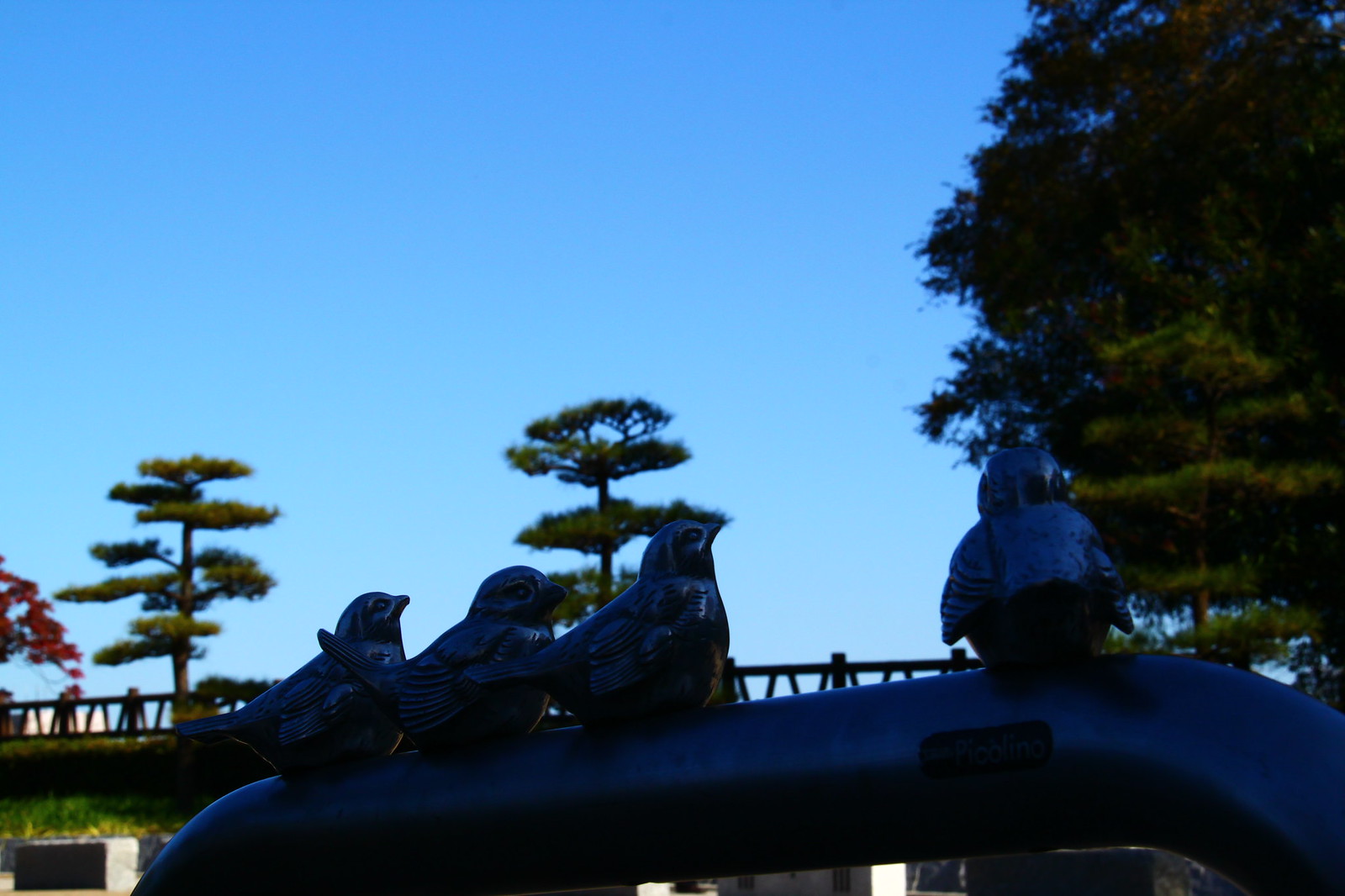In this realistic outdoor evening photo, the sky is a dark blue with whitish tones near the bottom and free of clouds, suggesting a sunset. The scene is somewhat blurred but shows significant detail. In the foreground, there is a black metal rail or banister, possibly part of a gate or fence, with four shiny, black bird statuettes. Three of these figurines are grouped together on the left, facing to the right, while the fourth stands apart, facing the background. To the left of the image, there is a tree with reddish leaves, partially out of the frame. Dominating the right side of the image is a large, green-leaved tree. In the background, a bridge with handrails is visible, indicating an elevated walkway. This bridge is framed by additional smaller trees, including a couple with green pine needles. The overall lighting is low, making it challenging to distinguish smaller details, giving the image a shadowy, serene atmosphere.